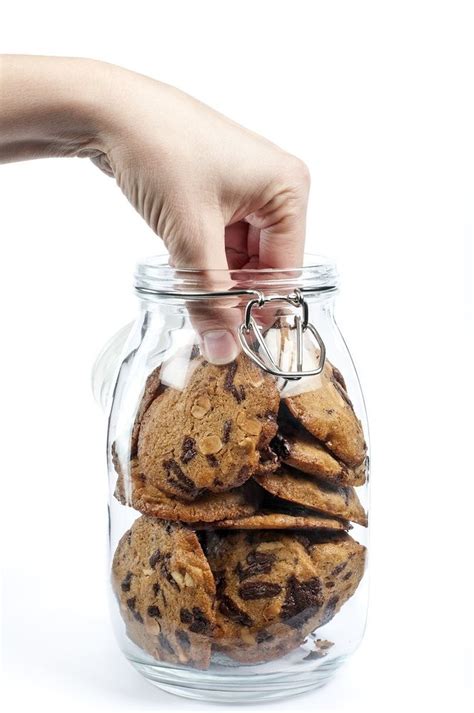The color photograph features a clear, round glass jar against a white background, filled to the brim with approximately a dozen chocolate chip cookies, some containing what appear to be nuts, possibly walnuts. The jar has an airtight metal clasp and a wire snap-on lid, which is seen hanging down to the left. A Caucasian hand with short nails is reaching into the jar, gripping a cookie from the top. The cookies inside are visually distinct, with dark chocolate chips and nut pieces scattered throughout, some arranged horizontally and others vertically.